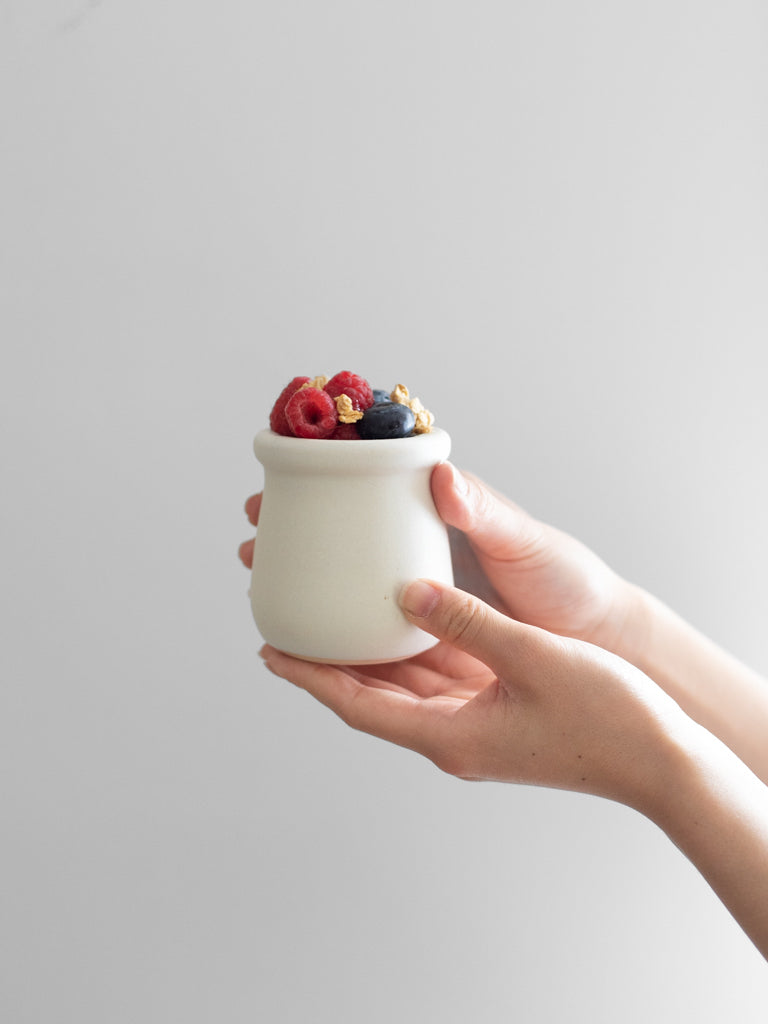In the image, there are two hands with very white, Caucasian skin, holding a white ceramic crucible filled with various berries. The hands emerge from the bottom right corner of the frame and lift the crucible to the center. The left hand supports the crucible from beneath, with the thumb balancing it in the front, while the right hand wraps around the back, with its thumb near the top and fingers visible along the outer edge. Inside the crucible, a few berries are visible at the top—red, circular raspberries, and darker, smooth berries that resemble grapes or blueberries. The background is a simple, light grayish off-white color, which enhances the focus on the hands and the crucible. There's also a slight reflection of light on the arms holding the crucible on the right side.